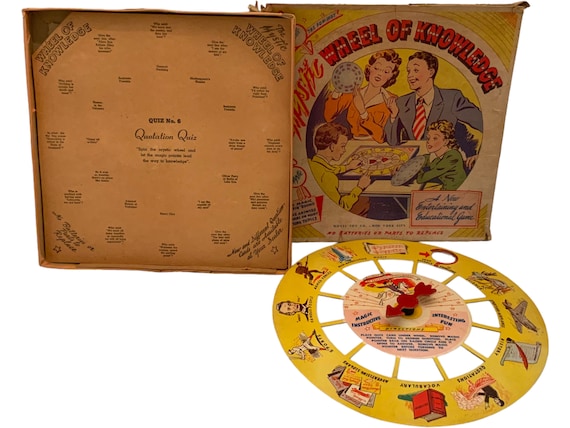The image depicts a vintage board game from the 1950s or 60s titled "Wheel of Knowledge," set against a white backdrop. The game features a brown, aged-looking foldable game board and a square box lid prominently labeled "Wheel of Knowledge." A circular yellow spinner with a red arrow occupies the bottom right-hand corner. 

The spinner’s perimeter showcases various images, including Abraham Lincoln, an airplane, a vocabulary book, a soldier, a baseball player, a series of books, and a scroll with a red feather quill, all surrounded by yellow spokes connecting to the central panel. This central area also hosts the arrow used to spin and select categories for gameplay.

The box lid displays a cartoon illustration of a 1950s-era family— a blonde mother in an orange dress with white trim, a father in a grey suit with a red and white striped tie, a daughter in a green dress, and a son with short brown hair in a yellow top—gathered around a table playing the game. The game contains elements prompting players to spin the wheel to receive categories and corresponding actions, as indicated by the red arrow in the spinner's center. Small black writing on the back panel further details the gameplay mechanics.